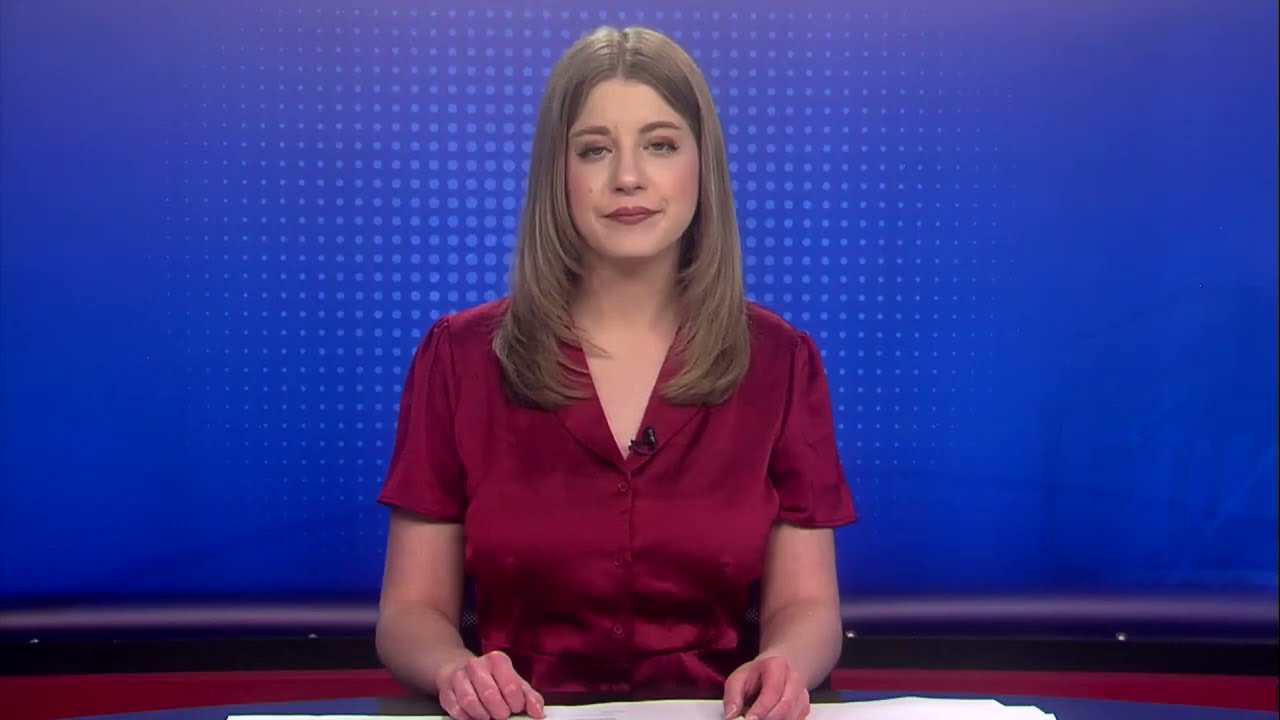This image captures a news anchor, seated at a desk covered in white papers, her hands rested calmly on the desk. She has a fair complexion and wears a dark red lipstick that complements her heavily blushed cheeks. Her long, straight light brown hair, which borders on dark blonde, cascades down to her chest, parted in the center and neatly tucked behind her ears, curving gently under her chin. Dressed in a silky, short-sleeved red button-up shirt, she sports a small black microphone clipped to her white collar. Her expression is neutral, with her mouth closed and her eyes giving a soft, heavy-lidded look. The backdrop is a blue screen adorned with light blue dots, enhancing the professional atmosphere of the news setting.